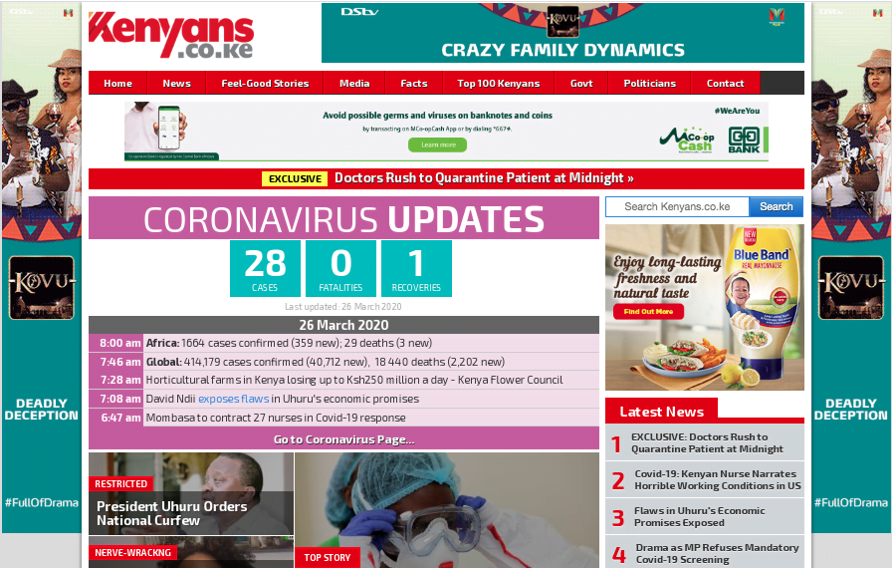The screenshot of the website is packed with content and various elements competing for attention. On the left-hand side of the image, two people sit down enjoying drinks; one is wearing a black hat and sunglasses, while the other, a female, dons a beige hat. Below them, to the right, is a sizable hashtag: "#WhiteIsDeadlyDeception," indicating some narrative or game full of drama.

The website has several navigational tabs at the top in red, with white text, labeled "Home," "News," "Feel Good Stories," "Media," "Facts," "Top Canyon," "100 Canyons," "Government," "Politicians," and "Contact." The banner next to this has the title "Canyons" in red, followed by the URL "engraved.co.ke."

In the content section, a white rectangle bordered in red and yellow bears the word "EXCLUSIVE" in black. Below it, a story flashes with the urgent headline, "Doctors rushed a quarantine patient at midnight." A purple border underneath heralds "Coronavirus Updates," with detailed statistics: "28 cases," "0 fatalities," and "1 recovery," indicating the data was last updated on March 26, 2020. Various timestamps such as 8:00 AM, 7:46 AM, 7:28 AM, 7:08 AM, and 6:47 AM with a purple background are indicative of real-time updates. 

Data specific to continents is presented: Africa has 64 confirmed cases, while globally, there are 414,179 confirmed cases. Additional content includes some local reports mentioning "Cultural farms in Kenya losing up to $250 a day," "David Nadi exposes flaws," and "Mom, that BASA took on contract 27 nurses and COVID response."

The website clearly aims to provide a comprehensive blend of news, updates, and additional stories, appealing to a diverse audience interested in current events, especially pertaining to the COVID-19 pandemic.